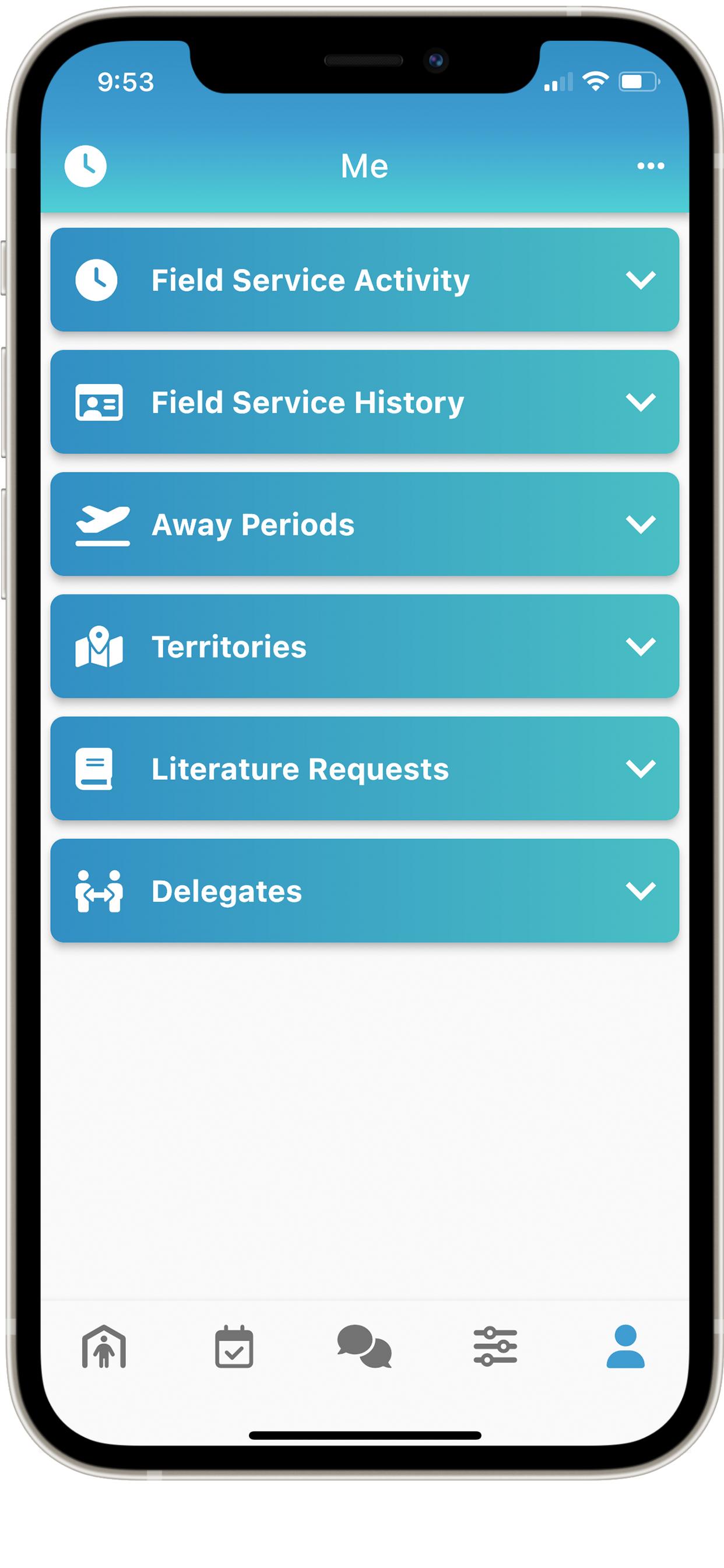Screenshot Description:

The image is a screenshot captured from a mobile phone. In the top-left corner, the time displayed is 9:53. Moving to the right, a Wi-Fi signal icon is visible, showing two bars filled in white, indicating a moderate connection strength. Adjacent to the Wi-Fi icon is a battery symbol, which shows the battery is slightly more than half full.

At the top of the screen, the label "me" is displayed, suggesting that this is the user's profile or a personal section. Below this, several drop-down menus are listed. The first menu is titled "Field Service Activity" and is accompanied by a watch icon. Following this, the next options are "Field Service History," "Away Periods" (which features an airplane takeoff icon), "Territories" (illustrated with a map icon), "Literature Requests" (indicated by a book icon), and "Delegates," which has an icon depicting two stick figures.

At the bottom part of the screen, there are additional navigation options, including a home button and a chat button, allowing the user to easily navigate the app or interface.